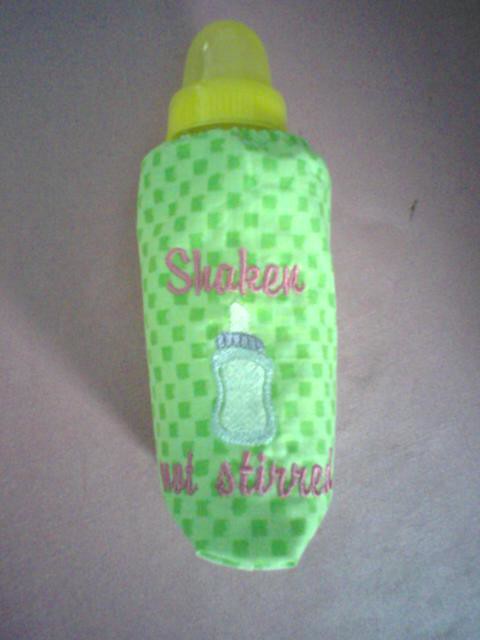In this overhead close-up photo of a baby bottle, the bottle is centered and adorned with a unique, eye-catching knitted sleeve, making it the focal point. The sleeve features a green checked pattern alternating between lime green and pale pastel green, concealing the bottle itself apart from its yellow lid and tip. Emblazoned on the sleeve in pink cursive script are the humorous words "shaken not stirred," with a blue knitted image of another baby bottle positioned prominently in the middle. The background appears to be a smooth white surface with a black scuff mark visible on the right-hand edge, contrasting slightly with the soft, cozy texture of the knitted bottle cover.